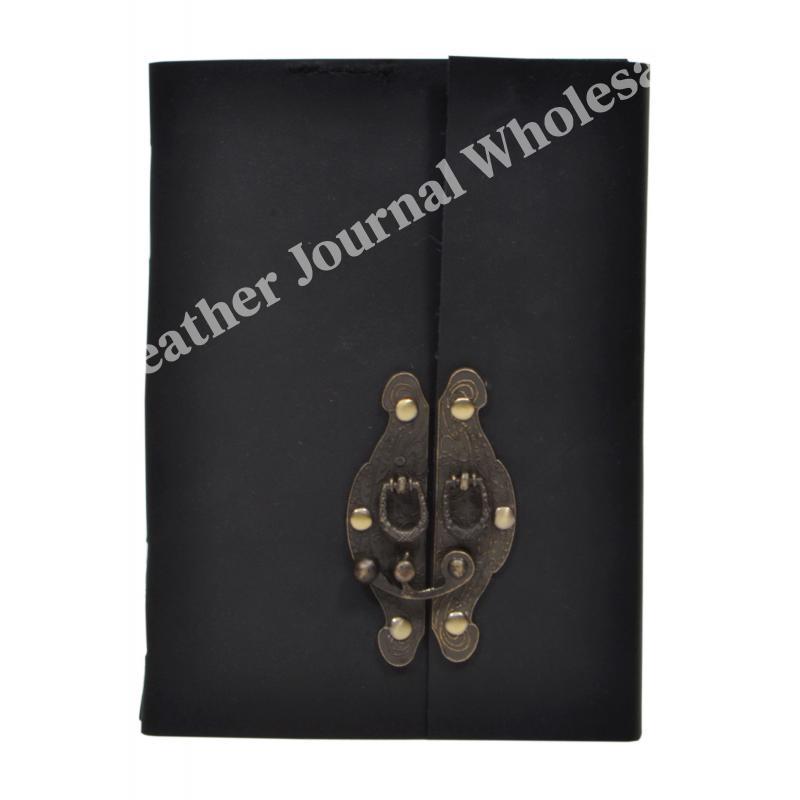This image showcases a close-up of a black leather journal cover, set against a white background with no visible borders. The cover, rectangular in shape and measuring approximately 5 inches tall by 3 inches wide, resembles a vintage binder that lawyers might have used for paperwork. The main feature is a metal clasp, made of brass and copper, secured by brass nails or studs. This clasp includes a curved latch that fits into a small round peg to keep the journal closed. About 1 inch from the top right and extending straight down is the break between the two pieces of the cover, indicating where it folds. In the lower third section of the cover, on either side of the split leather, are the metal latches. Diagonally across the upper portion of the cover, starting at the center left and moving towards the upper right, is the text "Leather Journal Wholesale" in light gray, almost translucent print. However, part of the text is cut off, displaying only "ather Journal Whole" before being obscured. This text suggests that the image might be an advertisement for a leather company.